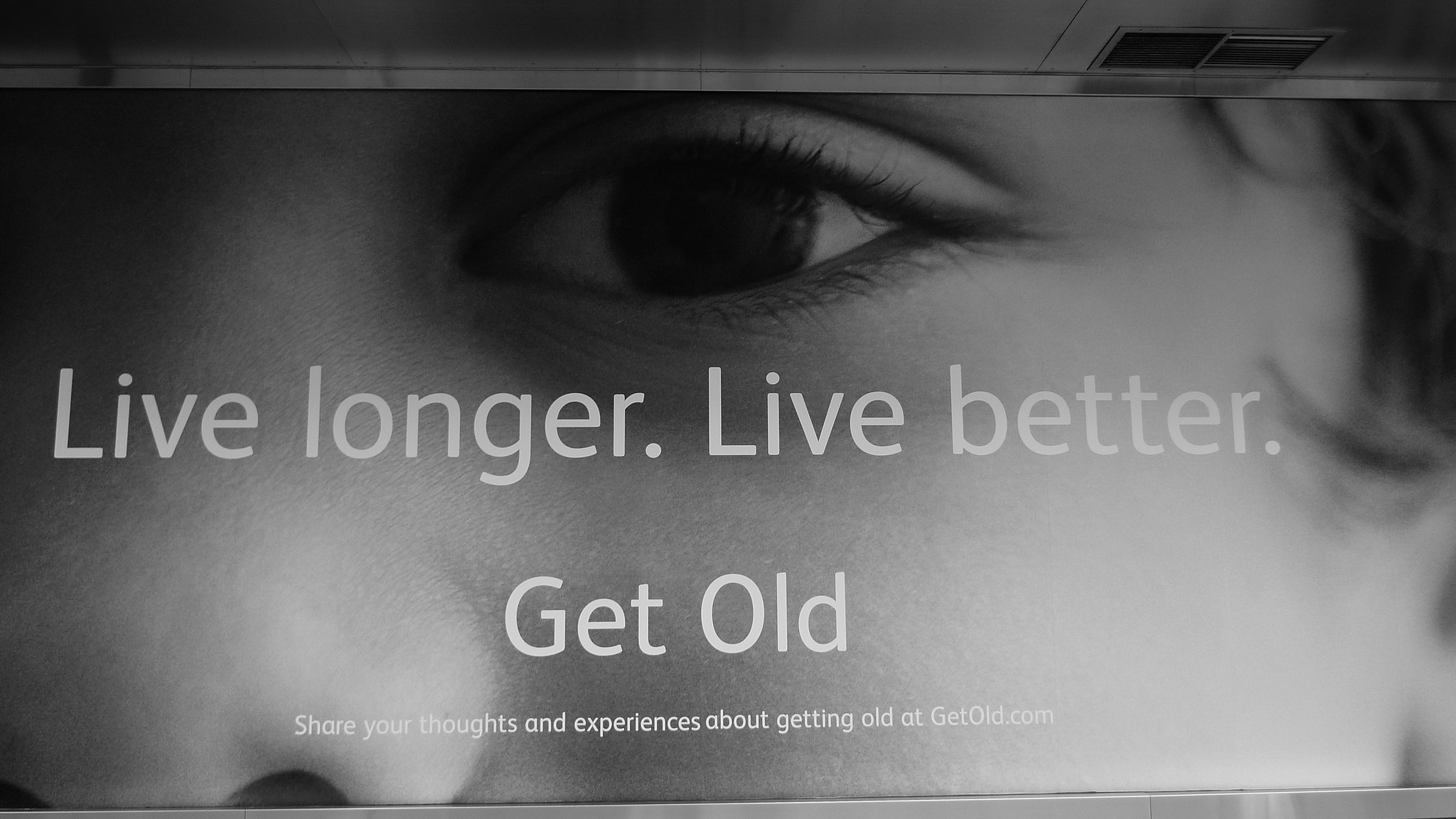This photograph captures a grayscale advertisement for a promotional campaign, likely positioned within a subway station, based on the metallic ceiling with visible vents and railings in the backdrop. The ad features a poignant black and white close-up of a child's face, focusing on the left eye, nose, and part of the cheek and hair. Dominating the center of the image is a message in bold white sans-serif font: "Live Longer, Live Better, Get Old." Beneath this main text, a smaller inscription invites viewers to "Share your thoughts and experiences about getting old at getold.com." The juxtaposition of a young child’s face with the topic of aging underscores the campaign’s focus on promoting healthy living throughout all stages of life.